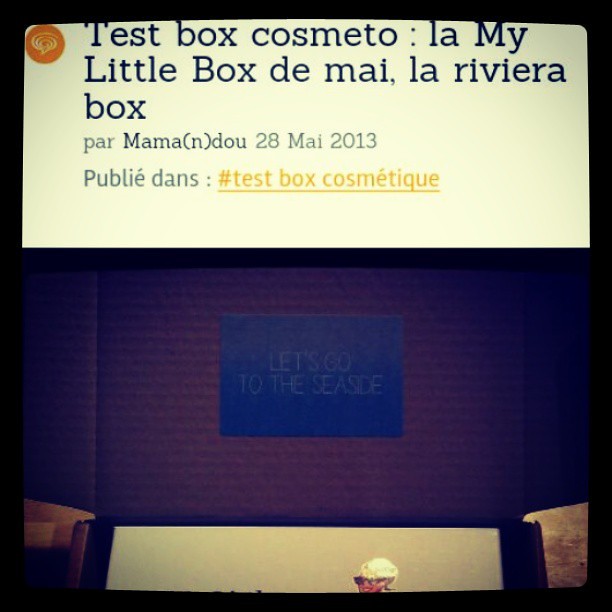The image appears to be a photograph of a computer or device screen displaying a slightly pixelated and darkly lit scene. At the top, clear typewritten text reads "Test box, Cosmeto, My Little Box de Mai, La Riviera Box par Mama (and in parentheses, an 'N'), 28 May 2013, Poublier dans Test Box Cosmetic." Below this text, a photo shows the inside of a box, predominantly dark but illuminating a blue plaque with the phrase "Let's go to the seaside." Beneath the plaque is a partial image of a woman with sunglasses, smiling. The inside of the box has indistinguishable details due to the darkness, although faint wooden structures are visible on both sides of the photograph. The whole image is bordered in black, giving it a framed appearance, with some color distortions including purplish-green hues and washed-out areas, adding to its enigmatic ambiance.